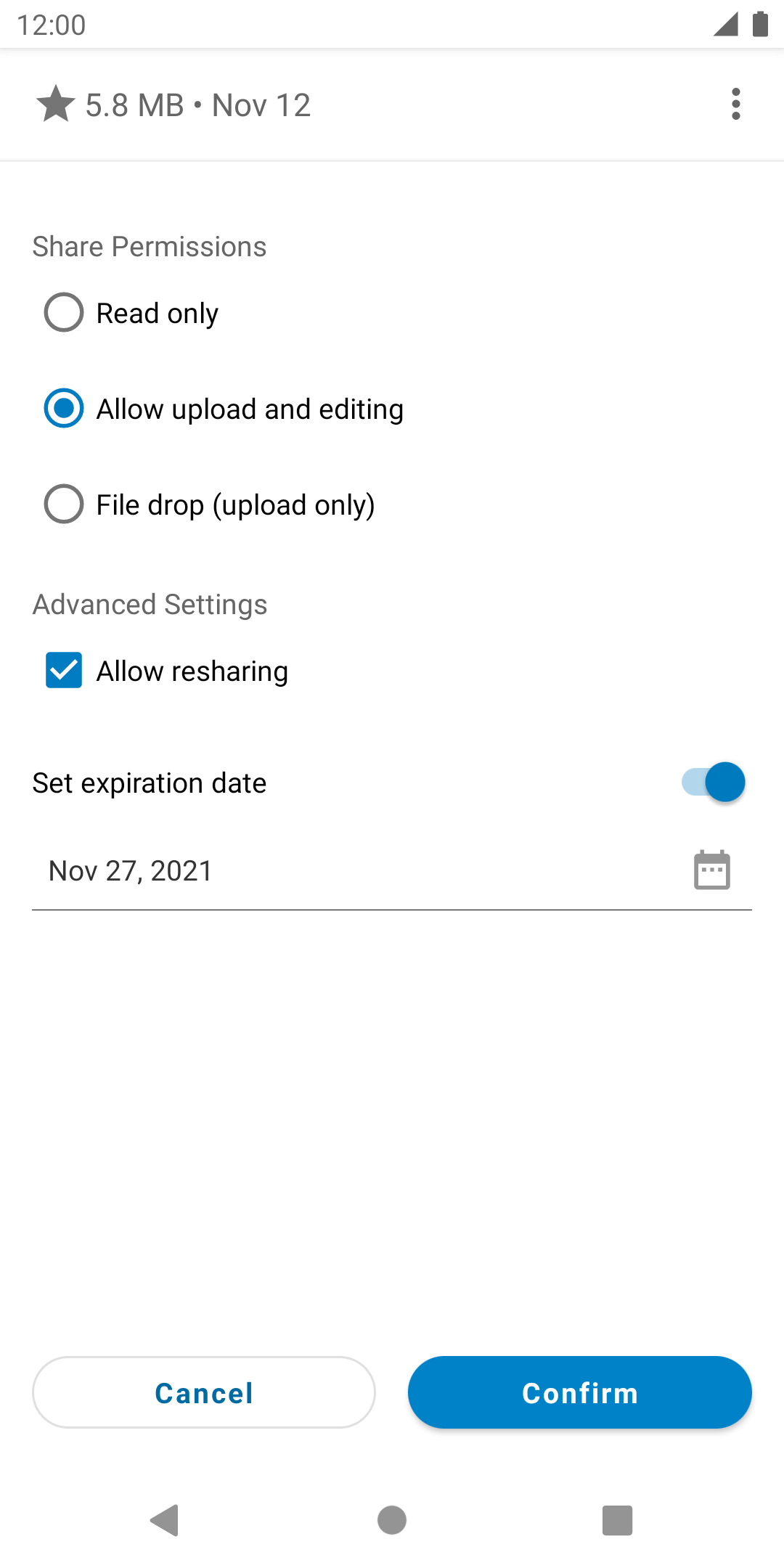The image is a detailed screenshot of a system settings page on a smartphone, observed at 12 o'clock with visible signal strength and battery power icons. At the top, indicative of the phone's status bar, are basic system indicators, including time, network signal, and battery life symbols.

Below this status bar is a section starting with "Star," followed by the text "5.8 megabytes, dot November 12th." Adjacent to this is a vertical ellipsis (three dots) icon, which unveils additional options upon interaction.

The options section begins with "Share permissions," accompanied by an empty white circle indicating the 'read-only' status. If selected, a blue dot would appear in the circle. Below this, an option with the blue dot already filled reads "Allow upload and editing," showing that it is currently selected. Another option beneath, labeled "File drop, upload only," displays an empty circle indicating it is unselected.

Further down is "Advanced settings," marked by a square which, when clicked, toggles a checkmark. This square is checked, indicating the "Allow re-sharing" option is active. There is also "Set expiration date," currently enabled, highlighting a specific date below it, "November 27th, 2021," accompanied by a calendar icon for date selection.

At the bottom of the screenshot, two action buttons are visible: "Cancel" and "Confirm," with "Confirm" highlighted in blue, implying it is the active choice. Finally, the standard Android navigation icons—a triangle, circle, and square—appear at the bottom, providing quick access to the phone's principal functions.